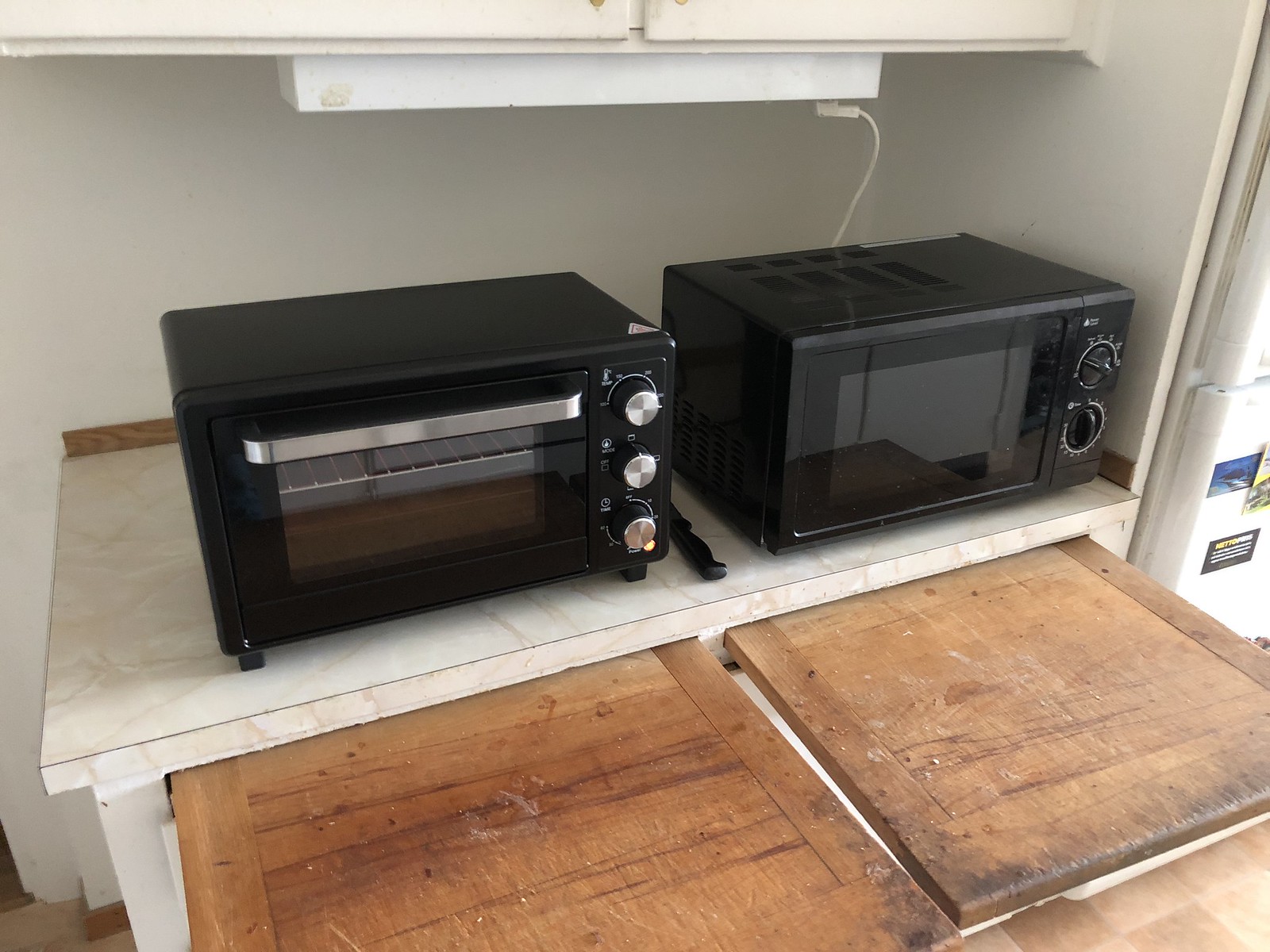The image depicts a cozy corner of a kitchen highlighting a large counter space with a creamy white Formica surface featuring faint, darker brown veining. On the left side of the counter sits a black toaster oven with a brushed metallic handle, a glass door, and three silver-topped dials situated on the right. To the right of the toaster oven is a black microwave, distinguishable by its two dials with white lettering. Positioned above this countertop is an off-white cabinet with a small fluorescent light fixture affixed to its underside, illuminating the workspace below. 

Beneath the counter are two medium brown wooden cutting boards that pull out, showing evidence of frequent use with numerous cut marks and slight staining. To the far right side of the image, part of a refrigerator is visible, adorned with several blue and gray stickers. The kitchen floor below is parquet, adding a warm texture to the area. This well-equipped corner offers both functionality and a cozy, utilitarian aesthetic.